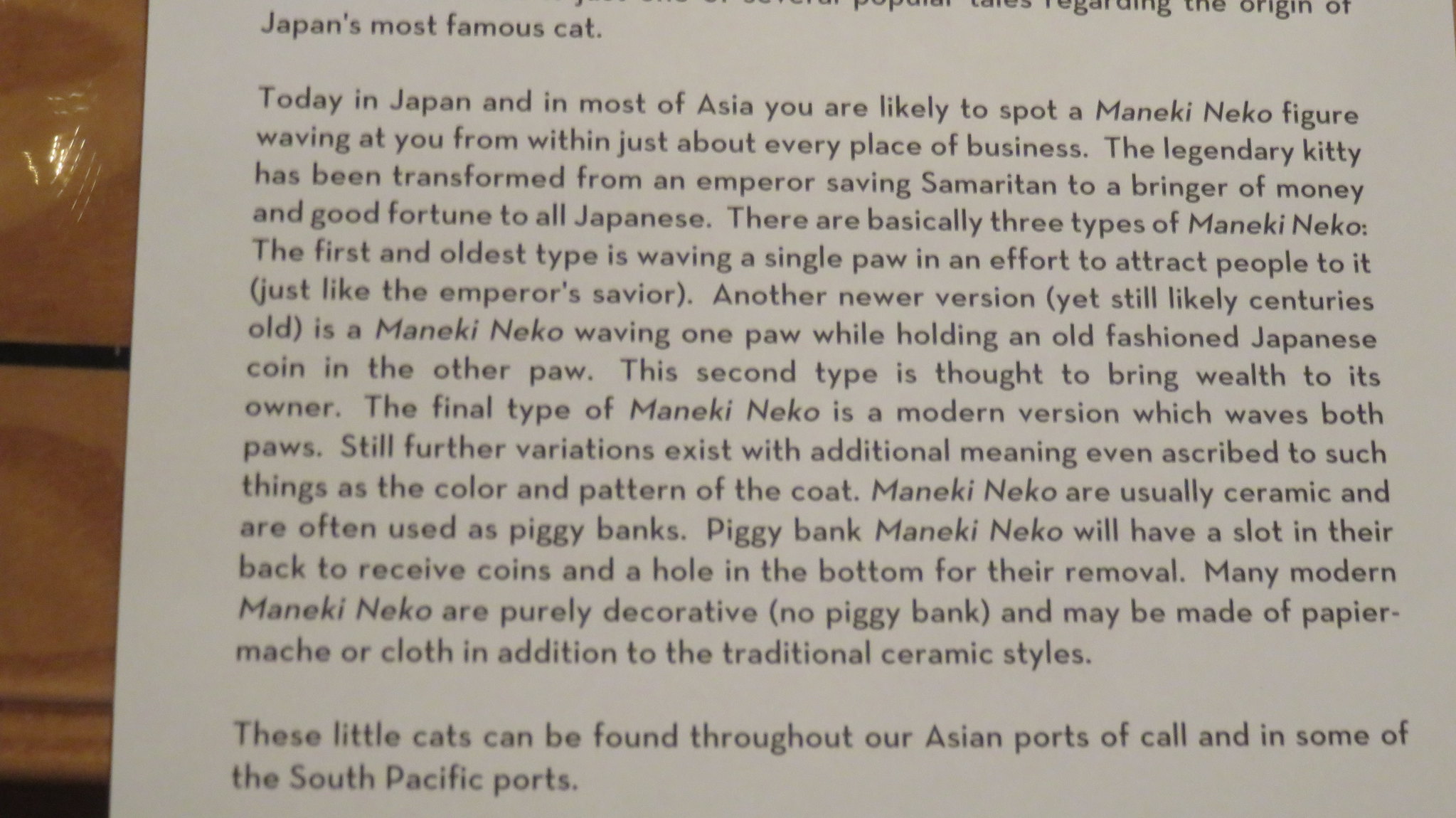In the image, there's a photograph of a white card displayed in front of a building or store, possibly against a window or on a table. The card features black text detailing the cultural significance of Japan’s most famous cat, the Maneki Neko. The sign reads: 

"Japan’s most famous cat, today in Japan and most of Asia, you are likely to spot a Maneki Neko figure waving at you within just about every place of business. This legendary kitty has been transformed from an emperor-saving Samaritan to a bringer of money and good fortunes to all Japanese. There are basically three types of Maneki Neko. The first and oldest type is waving a single paw to attract people, reminiscent of the emperor's savior. Another newer version, likely centuries old, features a Maneki Neko waving one paw while holding an old-fashioned Japanese coin in the other, believed to bring wealth. The final type is a modern version that waves both paws. Additional variations exist, with meanings attributed to the color and pattern of the cat's coat. Traditionally ceramic and often used as piggy banks, modern Maneki Neko can also be made from materials like paper mache or cloth and may be purely decorative. These little cats can be found throughout our Asian ports of call and some South Pacific ports."

This detailed description highlights the various types and cultural significance of Maneki Neko, while noting their widespread presence in business locations across Asia and other regions.